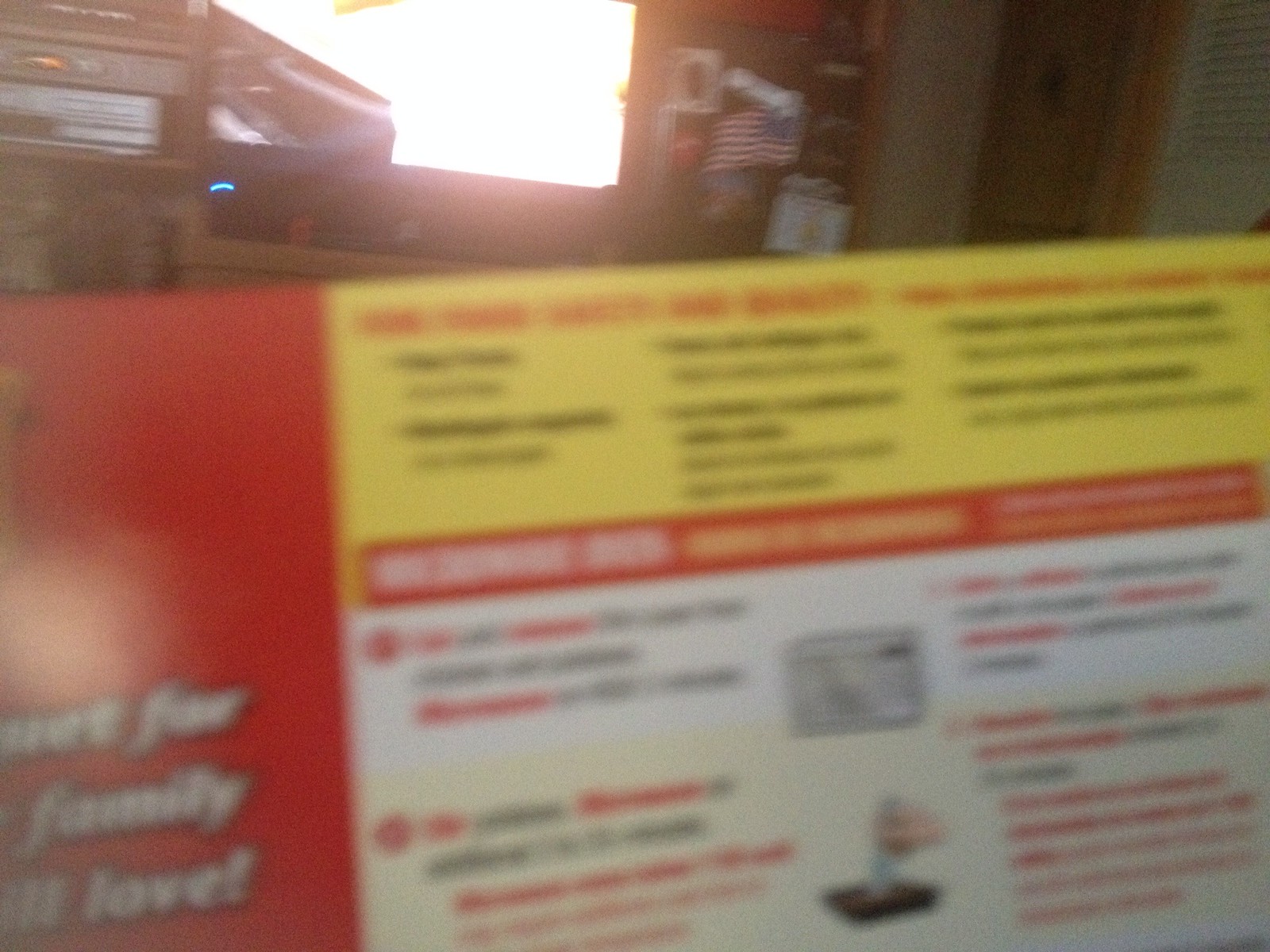This is an extremely blurry, close-up photograph of the back of a box, likely for a food product, taking up about 75% of the image. The left section of the box is red with barely legible white writing that hints at the words "family" and "love." To the right of the red section, the top quarter of the box spans horizontally in yellow with indistinct black and red writing. Beneath the yellow portion, there's a rectangular red strip with further white and yellow text. The bottom section is white with additional red and black lettering and features two indistinguishable illustrations, one of which possibly depicts a gray microwave, suggesting cooking instructions. In the background, a workspace with gray or tan walls is visible, along with a window to the left with light streaming through it and a small American flag to the right of the window. The entire scene is set against a blurry backdrop of indoor items.